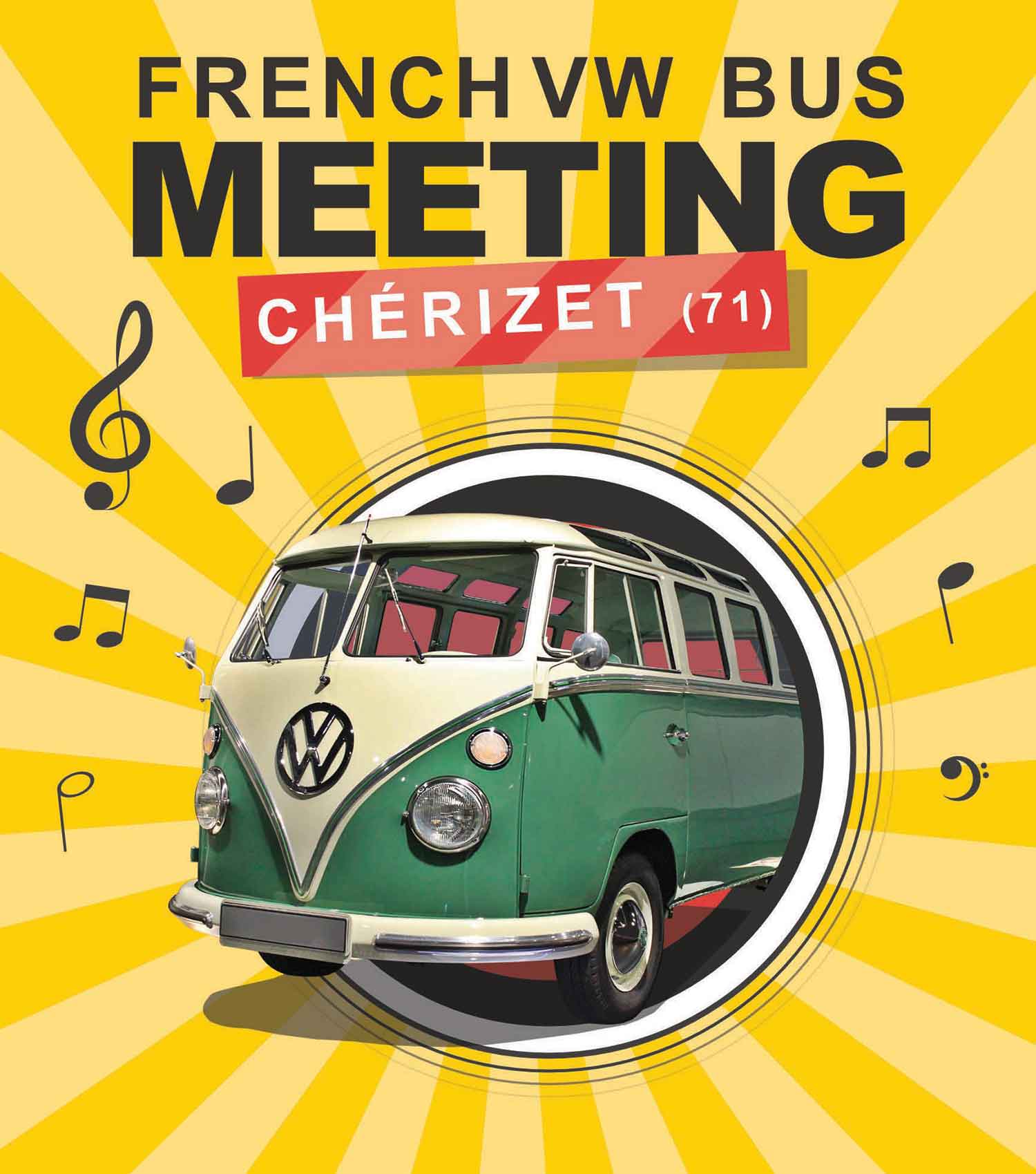The poster showcases a vibrant and nostalgic theme centered around a 1960s Volkswagen bus. At the top, "French VW Bus Meeting" is prominently displayed in bold black lettering. Below this, a red strip contains the word "Chérizet" with "71" in parentheses. The background is a radiant sunburst pattern with alternating stripes of light tan and yellow emanating from a central circle. Emerging from this circle is the front half of a classic VW bus, light green on the sides with a white front and the iconic VW logo prominently displayed. The bus, which appears to be coming out of a hole, is depicted with detailed features such as windows running down both sides and additional windows on the curved roof. Surrounding the bus are several musical notes, adding a playful and rhythmic touch to the image.